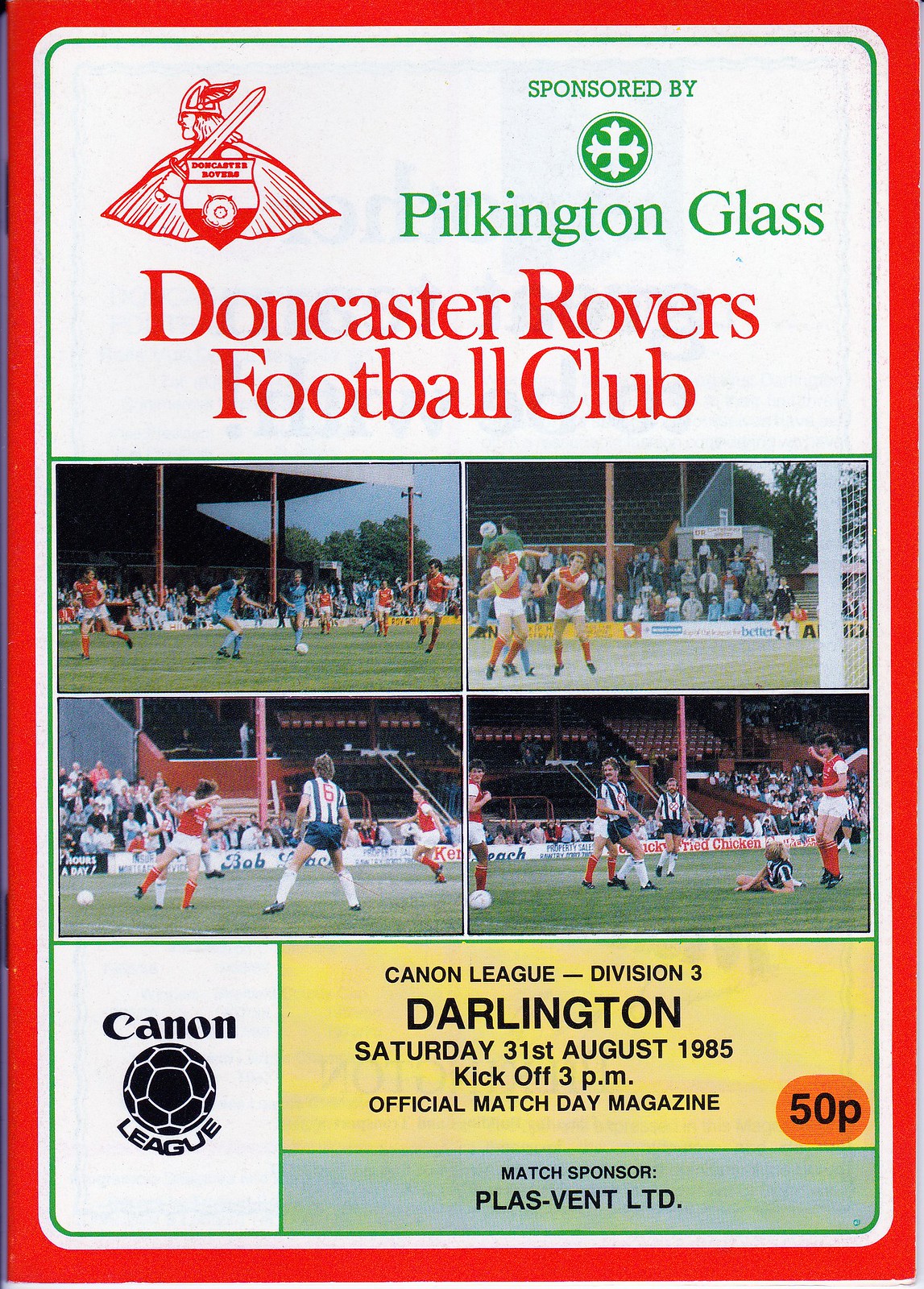The image depicts a full-color athletic event program from Saturday, August 31st, 1985, priced at 50 pence, for a soccer match featuring the Doncaster Rovers Football Club. The cover is primarily white with a striking red border and contains several elements arranged meticulously. At the top, bold red text reads "Doncaster Rovers Football Club," accompanied to its left by the team’s mascot logo: a red Viking-like figure holding a sword over his shoulder with a shield. Below this, green text states "sponsored by Pilkington Glass" along with the company’s symbol. Central to the cover, there are four distinct photographs in a two-by-two grid, each capturing moments from outdoor soccer games with players in red and white kits and spectators visible in the stands. Near the bottom, pertinent game details are presented in various text boxes. One red box highlights the game date and kickoff time, "August 31st, 1985, kickoff at 3 p.m.," while a green box states "match sponsor PLAS-VENT LTT." To the left, a logo for the Cannon Soccer League appears, indicating the competition's affiliation as Division 3. The design's organized layout and vivid color scheme make it an eye-catching and informative cover for the match day magazine.